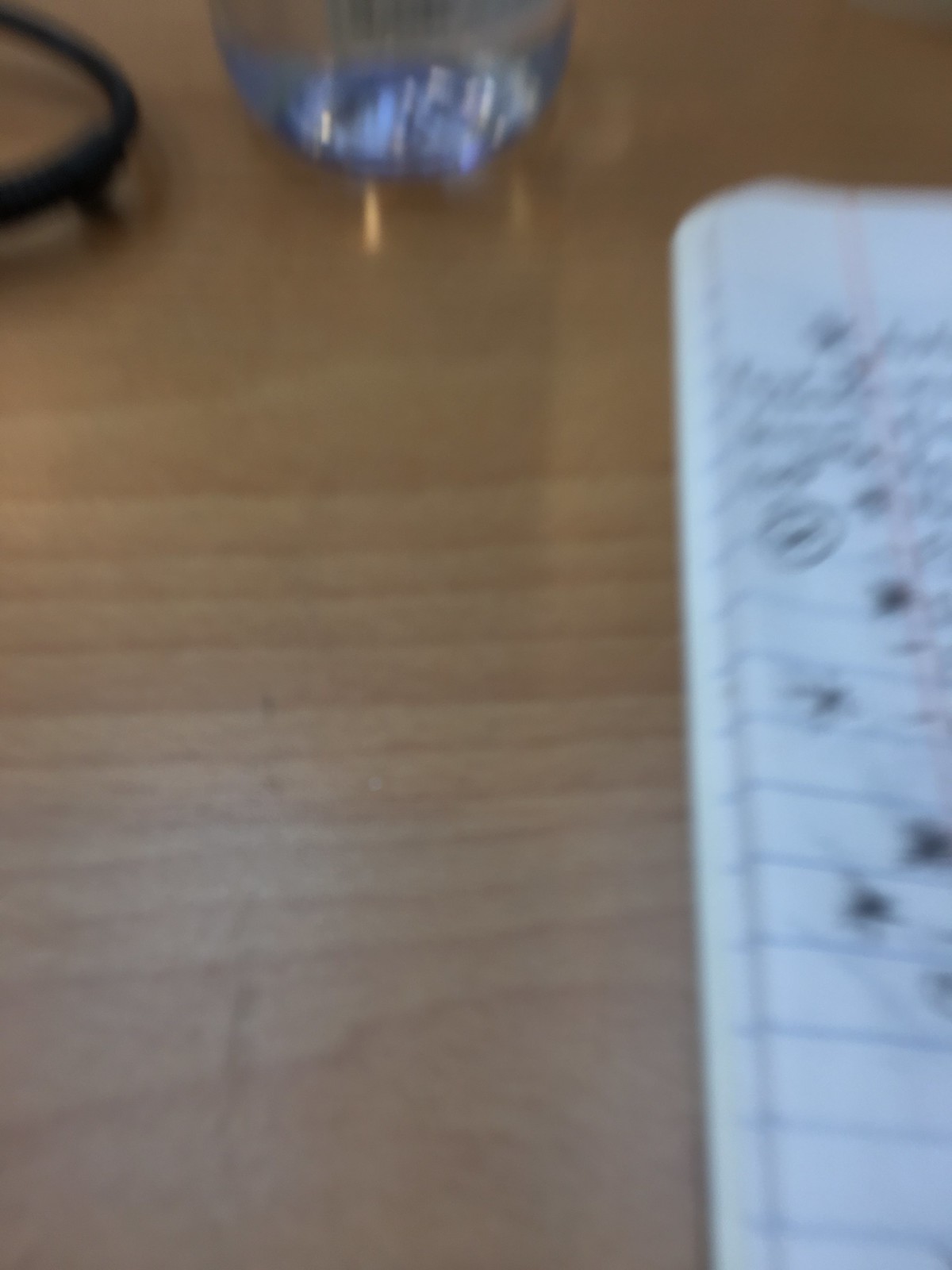The image captures a light wood grain tabletop with horizontal grain patterns. In the top left corner, there is a coaster featuring a black rim. Adjacent to the coaster, a glass object is visible; it is uncertain whether this is a drinking glass or a glass ashtray. Along the right side of the image, extending from the bottom to nearly the top, is a white notebook. Approximately a quarter of the notebook's page is visible, displaying some illegible handwriting.